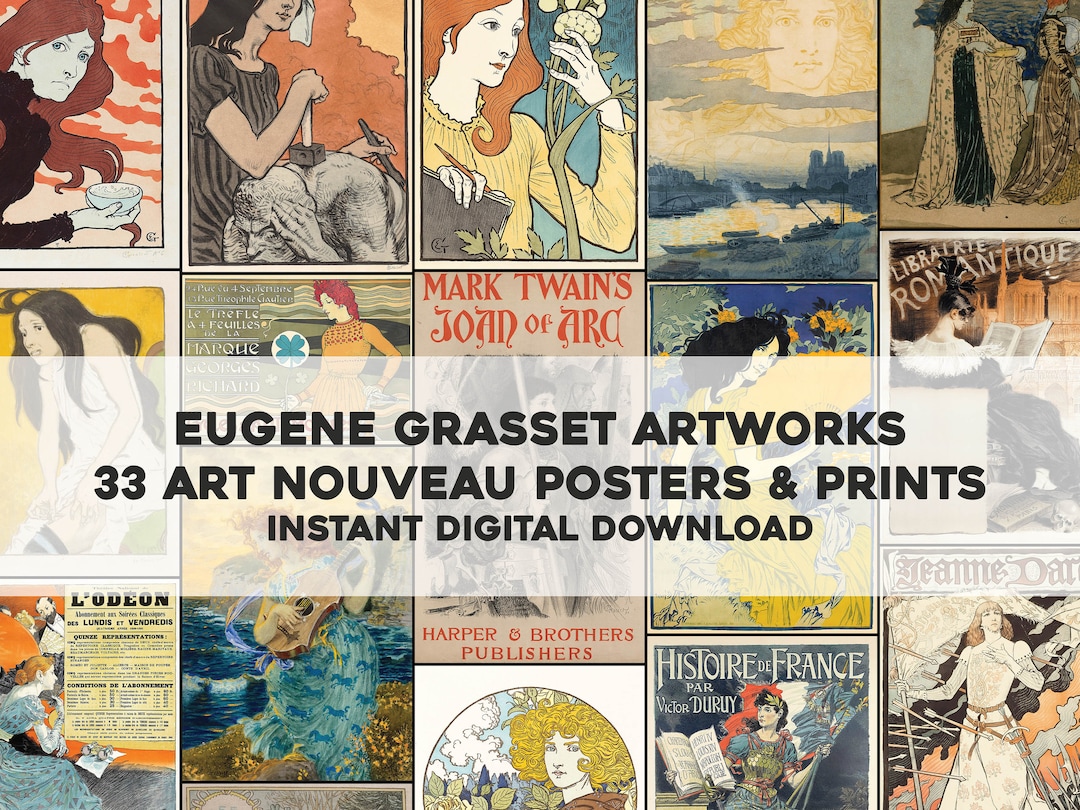The horizontal rectangular image displays a vibrant mosaic of Art Nouveau posters and prints, predominantly featuring women from various historical and cultural backgrounds, such as Joan of Arc and other French figures. Spanning the center of the image is a semi-transparent white band with bold black text that reads "Eugene Grasset Artworks," followed by the subtitle "33 Art Nouveau posters and prints" and the note "instant digital download" in smaller letters. The posters, showcased in a series of small rectangles, exhibit an array of themes and are indicative of a vintage yet classic French style. This image likely functions as an advertisement for a digital download service or an art collection.